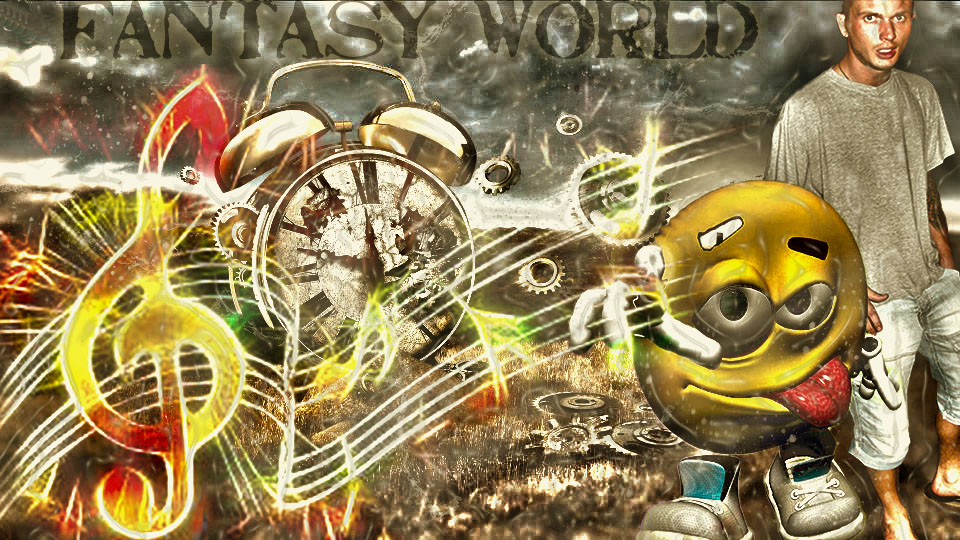The image appears to be an advertisement for a video game or app, characterized by its cluttered and colorful composition. At the top, in all capital black letters against a stormy gray, black, and white swirled background, the text "FANTASY WORLDS" is left-centered. On the right side of the image stands a barefoot young man, appearing serious, with the top of his head cut off from the frame. He is dressed in a grungy gray short-sleeved t-shirt and light blue capri pants. 

To his left, there is a distinctively whimsical animated creature resembling a silly Pac-Man. This creature features a large yellow face with a red tongue sticking out, asymmetrical eyes, and is adorned with oversized tennis shoes but no visible limbs. Further to the left of this creature, an old-fashioned, rusty gold alarm clock is present, with two bells on top and unreadable numbers due to the rust. Also situated to the left is a prominent red, yellow, and orange music note surrounded by wavy white lines extending across to the Pac-Man-like character. These musical elements further add to the chaotic and vibrant essence of the image.